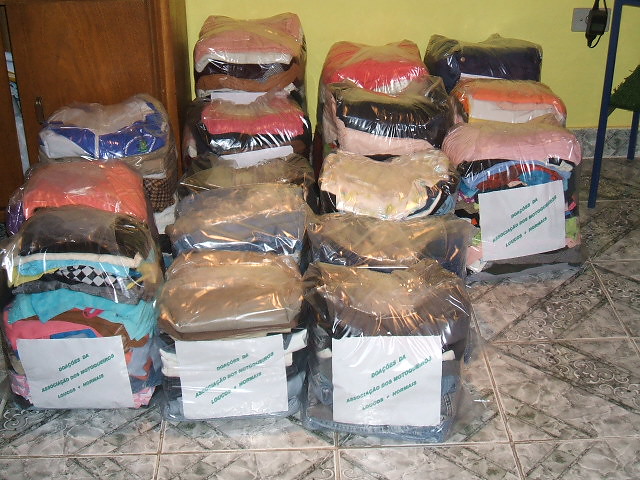The indoor color snapshot captures an organized array of approximately 15 transparent plastic-wrapped bundles of fabric or clothing lined up against a yellow wall. Each bundle features a white label with green, illegible text. The bundles, varying in height, contain a colorful assortment of items, including shades of pink, blue, orange, dark blue, white, brown, gray, and beige. They rest on a dark and light gray patterned tiled floor. In the upper left-hand corner, a brown cabinet partially comes into view. The items appear to be donations, potentially blankets or various types of clothing, ready for packaging and distribution. The setting suggests meticulous arrangement and preparation, hinting at an organized effort for aid or retail.